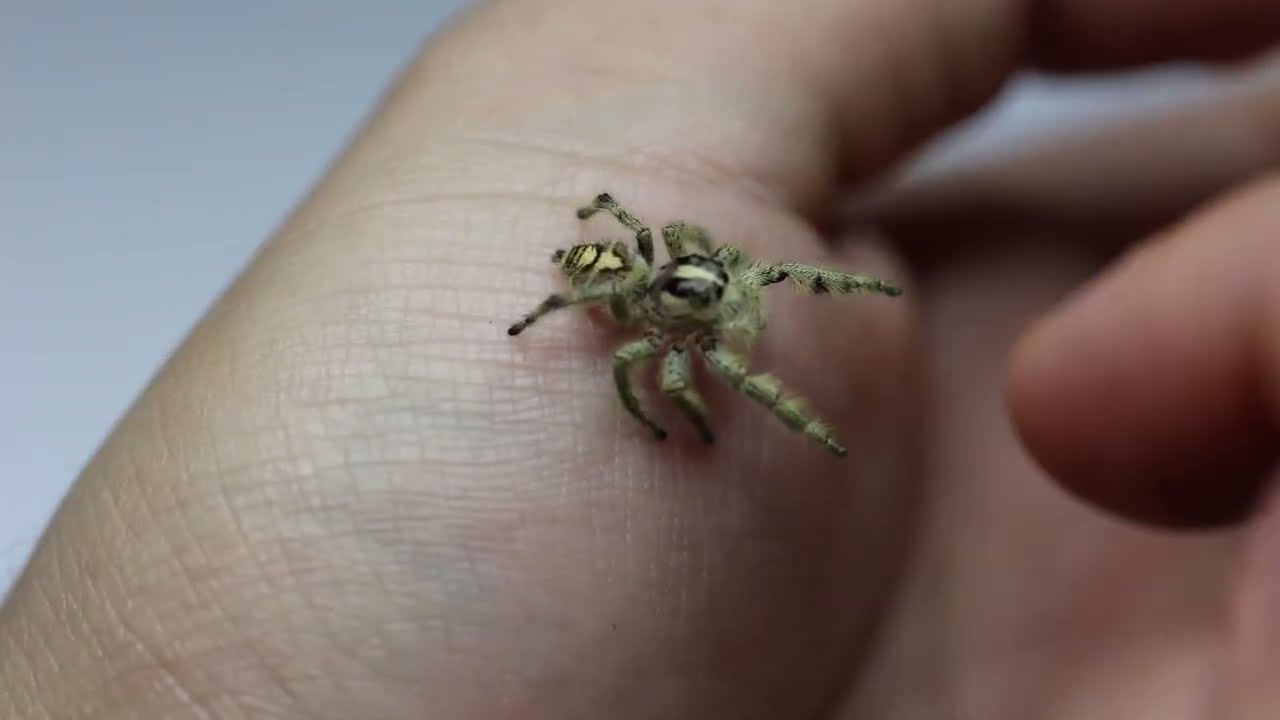The image features a highly detailed, close-up view of a person's left hand with a light blue, sparsely detailed background. The hand, palm facing up, occupies most of the frame, revealing the fine lines of the white skin in vivid detail. Fine lines and wrinkles are crisply visible, especially in the thenar eminence, the fleshy part of the palm near the thumb. In the foreground, a fingertip, probably the ring finger, is prominently displayed. 

Central to the image, perched on the thenar eminence, is a very tiny spider. The spider appears defensive, with its front two legs raised. It boasts a white, fur-like covering adorned with black and yellowish-tan markings. Despite its minute size – suggested to be smaller than a dime – the spider stands out sharply against the skin of the hand. Its gold-accented body and eight fuzzy legs, complete with black spots and stripes, add to the intricacy of this macro shot.